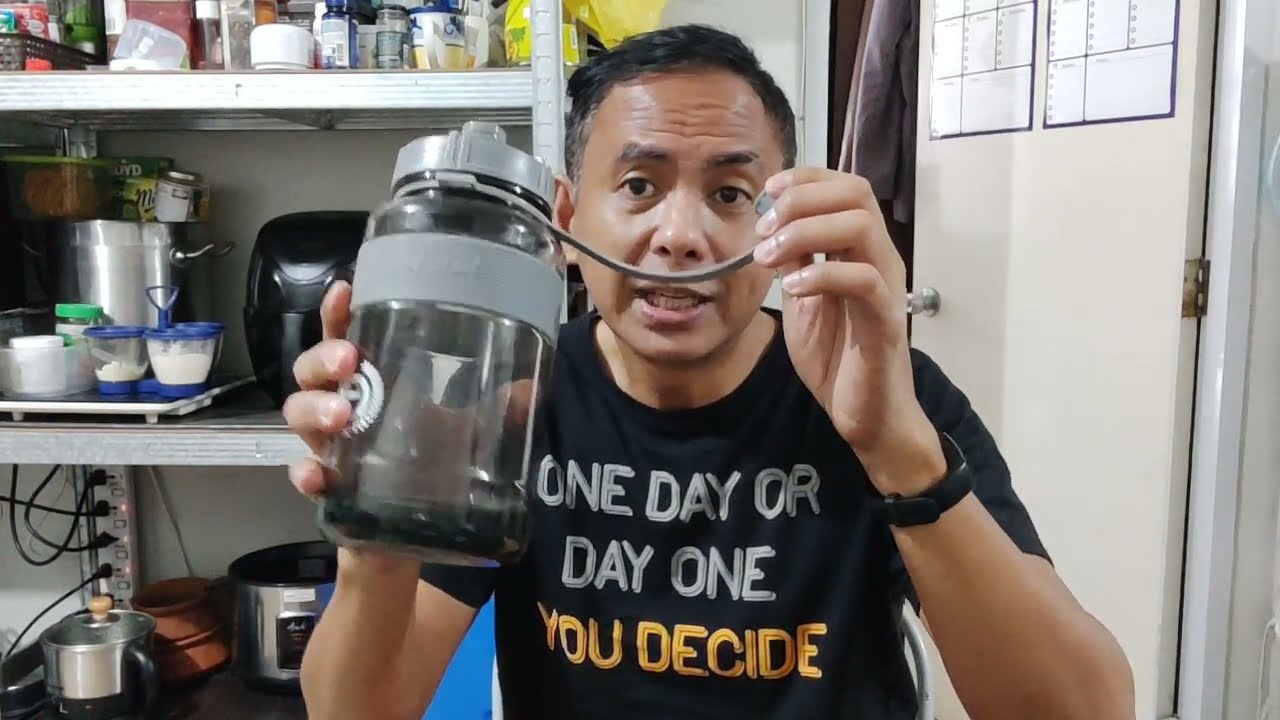The photograph depicts a middle-aged man of Asian descent, captured indoors. He is seated and talking energetically to the camera, suggesting he might be recording a video. The man has tan skin, short black hair graying at the sides, disheveled eyebrows, almond-shaped eyes, a slightly flat nose, and pink lips. He is wearing a black t-shirt that features the motivational text "One Day or Day One" in light gray letters, followed by the phrase "You Decide" in yellow letters. His left hand is raised, holding a gray and black plastic water bottle, while his right hand holds the detached lid, connected by a plastic tether. The man also wears a black wristwatch on his left wrist. Behind him, on his left, there are metal shelves stocked with kitchen items, and on his right, there's an open off-white door leading to another room, possibly featuring a closet since a jacket can be seen hanging in the background. His eyebrows are slightly raised, with furrows on his brow and wrinkles along his forehead, adding to his expressive demeanor.